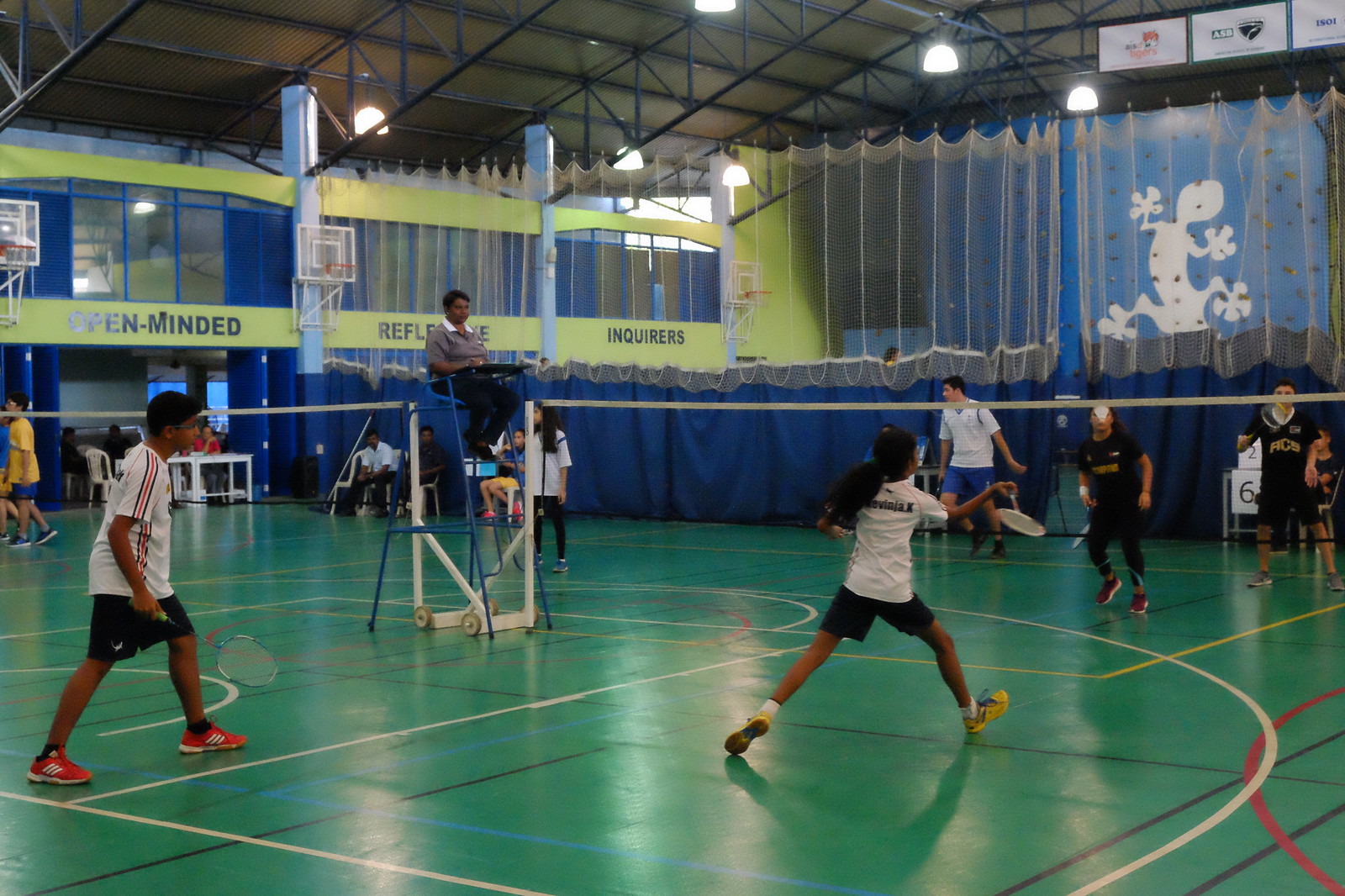In a large, vibrant gymnasium with a blue interior divided by a big curtain, an energetic badminton scene unfolds. The spacious venue, featuring greenish floors marked with game lines and visible trusses and lighting fixtures, hosts multiple badminton matches simultaneously. Basketball hoops can also be spotted in the background. The focal point is a lively doubles match. At the forefront, a young girl, donned in a white shirt, black shorts, and yellow shoes, is captured mid-action, about to hit the shuttlecock back to the opposing team. Her partner, a young boy in matching attire but red shoes, stands by her side. Their opponents, dressed in all-black uniforms, are poised across the net, with one wearing white shoes and the other in red. Overseeing the game from a tall ladder bench is a referee in a gray shirt with a white collar, black pants, and black shoes. A few spectators, predominantly appearing to be of Indian descent, along with diverse onlookers, observe the match intently from the background. An official in a white shirt stands further back, enhancing the organized atmosphere of this spirited event.